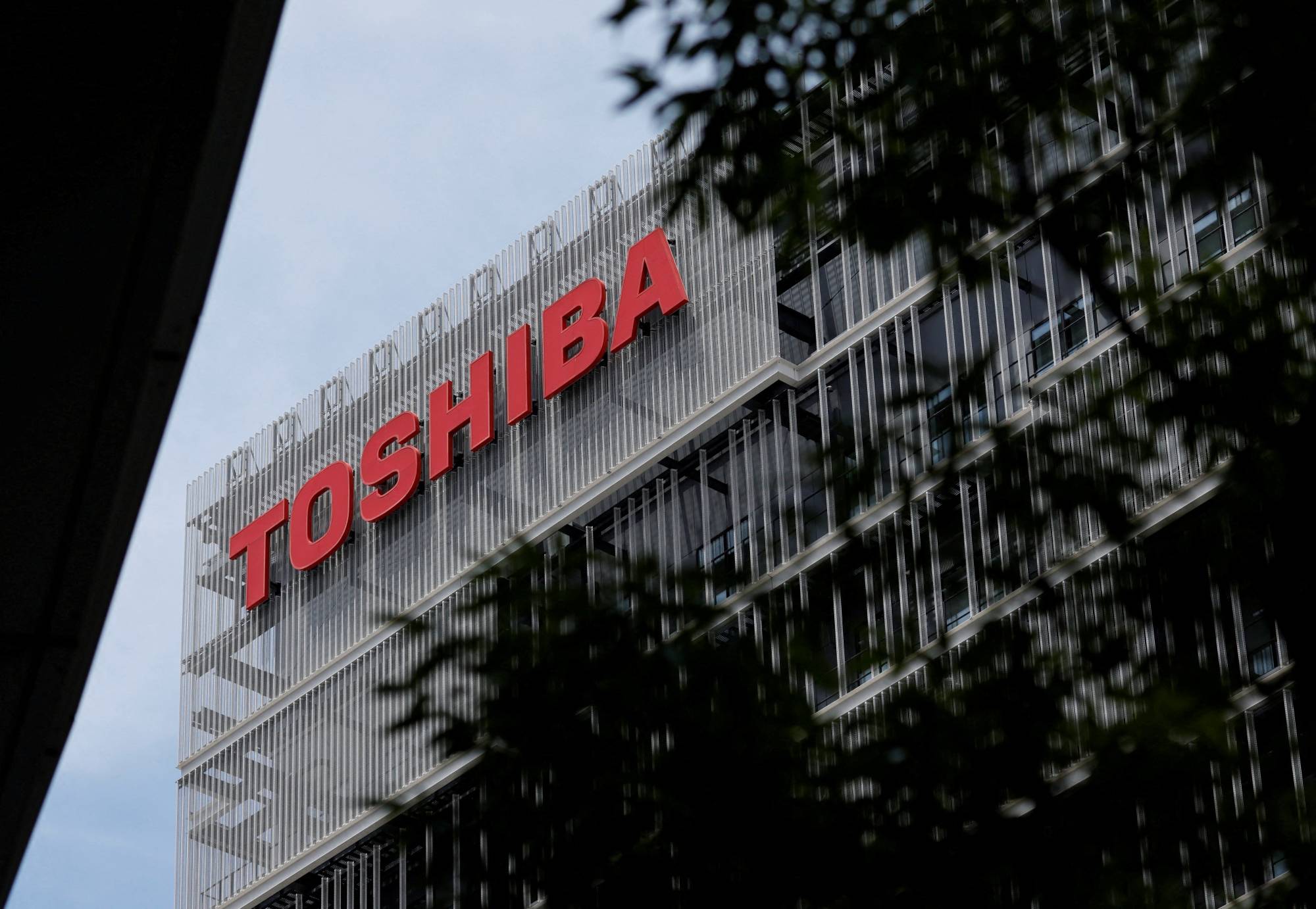This photograph, taken in daylight, captures a close-up, low-angle view of a large, modern office building adorned with large, bold red letters spelling "Toshiba" near the top of its face. The perspective implies the photographer was almost lying on the ground, aiming the camera upwards through some tree branches that cast shadows on the sleek, black metal and steel structure. The windows, long and angular, add to the modern aesthetic of the building, which features stainless steel tubing or poles along its sides, hinting at some functional architectural design. The sky above is light blue with scattered clouds, suggesting a bright yet slightly overcast day, evocative of a vintage photograph from the early 80s or 90s.